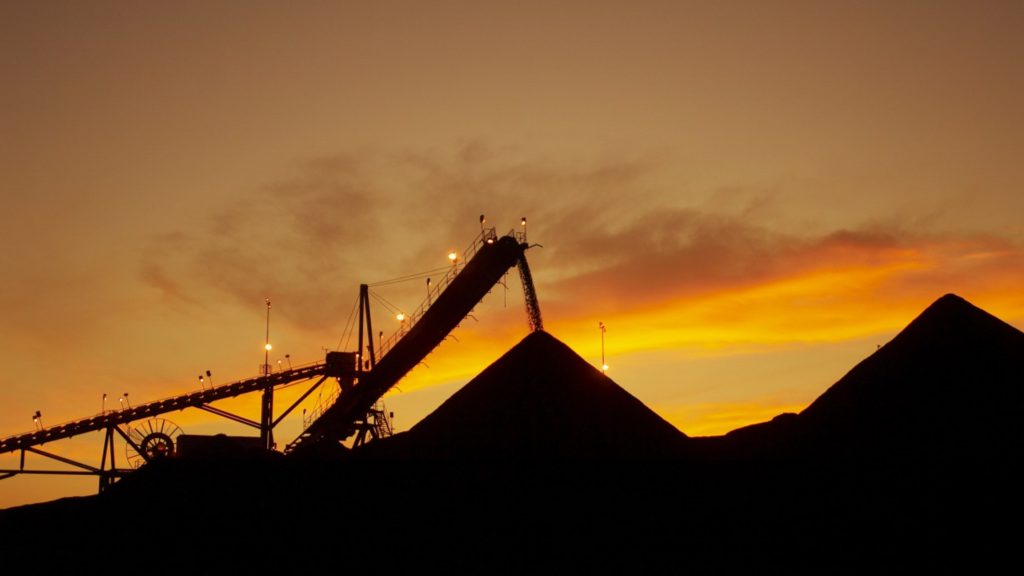This color photograph captures an expansive industrial mining site silhouetted against a breathtaking sunrise. Dominating the composition is the striking sky, transitioning from a deep mauve at the top to radiant yellow near the horizon, accented with swirls of orange and yellow clouds. Along the left side, a large conveyor belt, illuminated by lights, stretches diagonally upward from the foreground to a towering metal structure reminiscent of a derrick. This conveyor is in the process of dispensing material, likely gravel or ore, onto one of two prominent pyramid-shaped mounds below. The right side of the image is anchored by another mound, standing stark and solitary without any visible machinery nearby. The entire scene, bathed in the golden hues of dawn, creates an ethereal landscape of industrial silhouettes against a glowing sky.